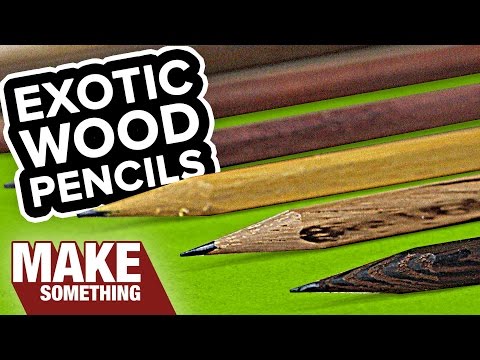The image, likely a screenshot from a YouTube video thumbnail, shows a neatly arranged row of several wood pencils on a green surface. The pencils are displayed in a gradient of colors starting from the top: reddish brown, yellow, light brown, and dark brown. Each pencil's sharp black nib points to the left. Overlaying the top left of the image are the words "Exotic Wood Pencils" in large, white capital letters within a black area. At the bottom left, "Make Something" is prominently displayed in white text on a bold red background. The image is framed by black bars on the top and bottom, enhancing its polished look. The pencils appear unique and are not the typical variety found in everyday stores.